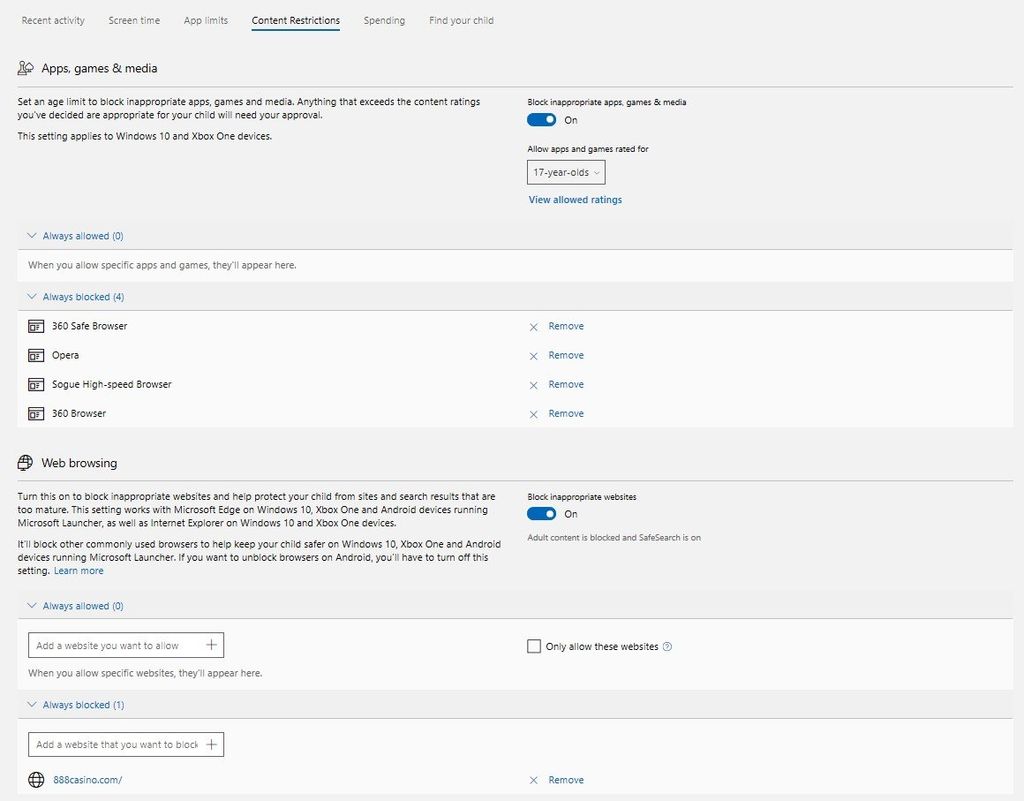The image depicts a parental control app allowing parents to set various restrictions on a child's digital activity. Specifically, the "Content restrictions" tab is selected, highlighted in bold black letters with a blue underline beneath. Other available options include "Recent activities," "Screen time," "App limits," "Spending," and "Find your child."

Under the "Content restrictions" section, parents can set age limits to block inappropriate apps, games, and media. The text explains that any content exceeding the predefined ratings will require parental approval, and this setting is applicable to Windows 10 and Xbox One devices. There is an option to block inappropriate apps, games, and media, which is toggled on with a blue button. The permissible rating is set for apps and games suitable for children aged 4 to 17 years old.

In the "Always allowed" section, parents can specify apps and games that will always be permitted, although no specific items have been added here. 

The "Always blocked" section lists several pre-blocked browsers: 360 Safe Browser, Opera, Soak High-Speed Browser, and 360 Browser. These have the option to remove them indicated by an "X" and the word "Remove" next to each.

Underneath, the "Web browsing" section is set to block inappropriate websites, a feature that is currently turned on. There are no websites listed under "Always allow," indicating no exceptions have been made. However, under "Always blocked," the website 888casino.com is specifically mentioned as blocked.